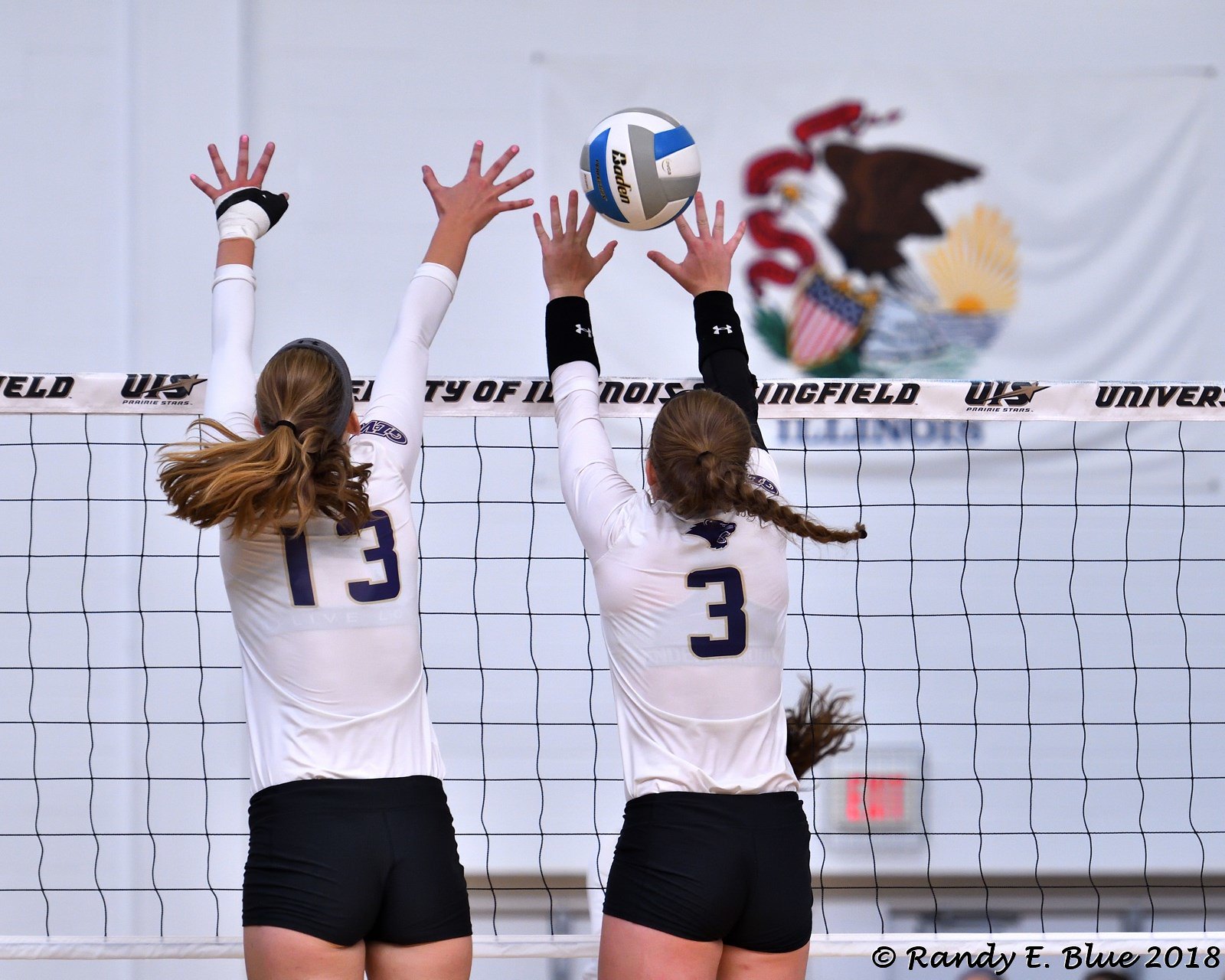In this dynamic image capturing a volleyball game, two women are at the center, leaping to block a ball. Their backs face the camera, and they are both clad in white long-sleeve jerseys and black shorts. Both women have long brown hair, with one in a braid. The player on the left is wearing jersey number 13, while the one on the right dons jersey number 3. They both have their hands extended high above the net, fingertips spread wide, aiming to intercept a white volleyball adorned with blue and gray lines. The net in front of them partially obscures a logo that reads "University of Illinois Springfield" (UIS). Behind them, a white wall features a blurred banner with a multicolored design, adding to the atmosphere of the sporting event. The image is credited to Randy E. Blue, 2018, as noted in the bottom right corner.